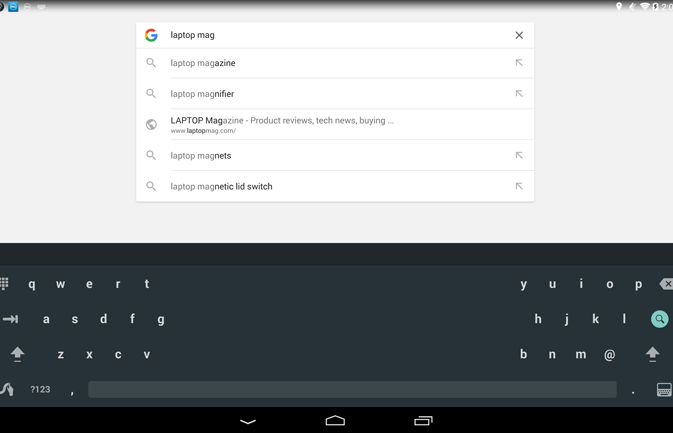This image is a screenshot of an unidentified web page, set against a clean, white background. Prominently displayed at the top is the Google icon, followed by an assortment of text related to "Laptop Mag." These include: "Laptop Magazine," "Laptop Magnifier," "Laptop Magazine, Product Reviews," "Tech News," and the URL - "www.laptopmag.com." Additional lines read "Laptop Magnets," and "Laptop Magnetic Lid Switch." Dominating the bottom part of the image is a black keyboard with white letters. Notably, there is a significant gap between the 'QWERT' section on the left and the following 'YUIOP' keys on the right, indicative of a split or ergonomic keyboard design. The scene is devoid of any living beings, such as people, animals, birds, or vegetation, nor does it feature any architectural elements, vehicles, or bicycles.